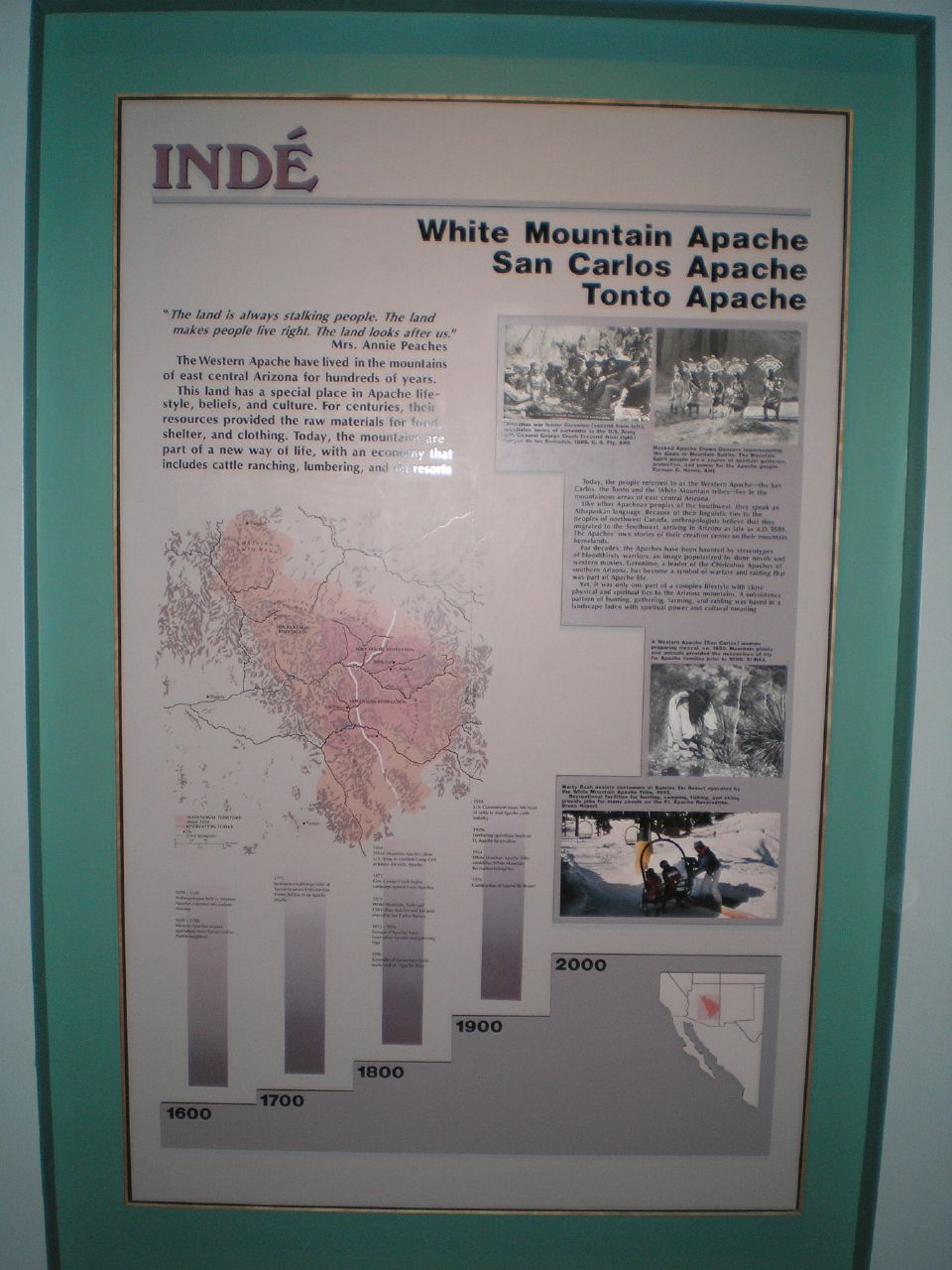The image is a framed infographic, featuring a teal green border and a central white panel with a gold accent. The top section prominently displays "INDE" in capital letters, followed by the names "White Mountain Apache," "San Carlos Apache," and "Tonto Apache." At the heart of the infographic is a meaningful quote from Mrs. Annie Peaches: "The land is always stalking people. The land makes people live right. The land looks after us." Below the quote, detailed text describes the Western Apache's historical and cultural connection to the mountains of East Central Arizona, highlighting their long-standing practices and contemporary adaptations. The land has provided essential resources for food, shelter, and clothing for centuries, and continues to play a role in modern activities such as cattle ranching, lumbering, and resort operations. The infographic is further enriched with black-and-white photographs depicting Apache individuals, a color-coded map of the region, and a timeline bar graph spanning from 1600 to 2000, illustrating significant temporal data about the landscape and its population.